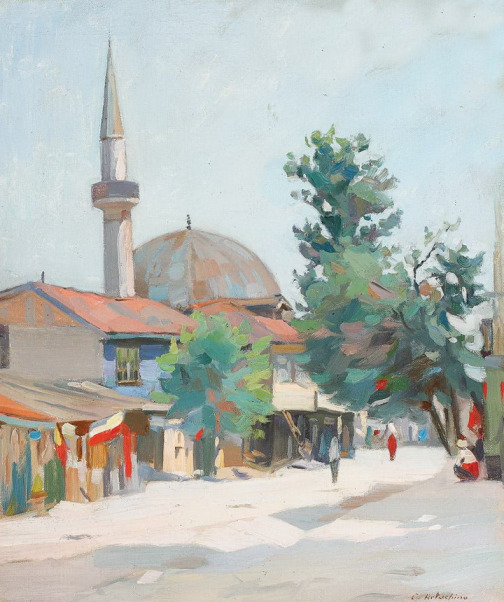This painting portrays a vibrant street scene in what appears to be a town reminiscent of places like India. Dominating the background is a majestic building with a large, curved dome and a very thin, pointed tower beside it, featuring a turret or balcony near the top. This building might be a mosque or temple, adding an exotic charm to the setting. In the foreground, there are several low-rise, colorful buildings, perhaps houses or merchant shops, with a significant tree on the right-hand side. A man is sitting under this tree, and a few people are either squatting or walking along what seems to be a dirt road. Their indistinct forms and the painterly, impressionist style render them almost shadow-like. The scene is bathed in daylight, with shadows of the trees cast on the sandy-colored ground. The sky above is a pale blue with light clouds, contributing to the overall pastel brightness of the painting. The impressionist technique and the vibrant, detailed depiction of everyday life offer a striking, picturesque view of this foreign town.